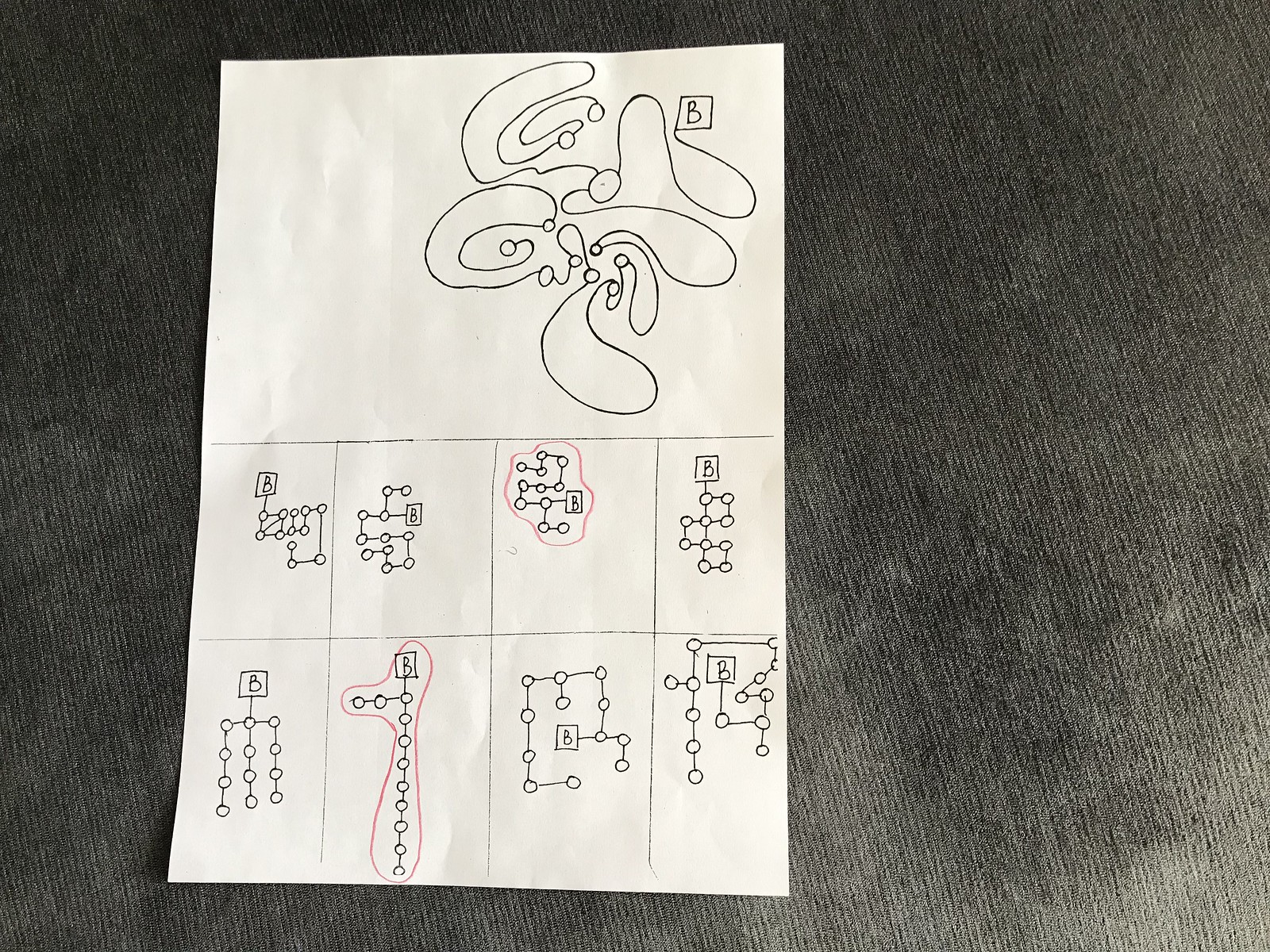The photograph captures a white piece of paper resting on a dark gray, cloth-textured surface. The surface has a vertical texture, gradually lightening towards the bottom of the image. The paper itself appears slightly crumpled, with subtle folds indicating it had been handled previously. 

The paper is divided into two sections. The top half features a larger, hand-drawn image created with black pen. This drawing consists of a series of squiggly lines interspersed with circles. In the top right corner of this drawing, there is a square containing the letter "B."

Below the larger image, the bottom half of the paper showcases a grid of eight smaller images, each enclosed within its own small rectangle. These drawings primarily consist of straight lines connected by circles at each junction, where bends occur in the design. Notably, two of these smaller images are encircled in red, likely drawn with colored pencil, highlighting them distinctly from the others.